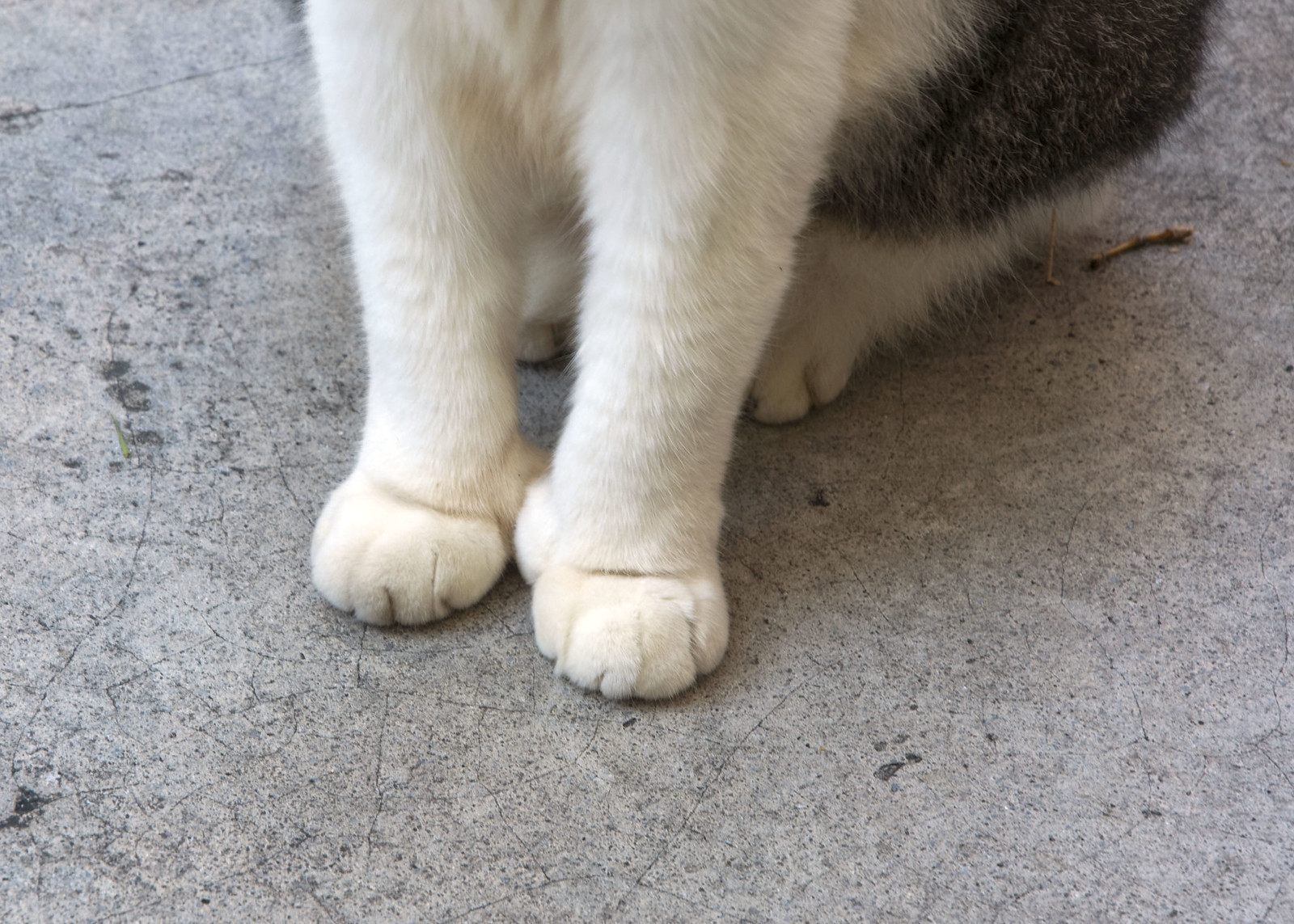This color photograph captures the lower half of a cat, from the chest down, positioned on a cracked pavement. The pavement exhibits variations of black, white, and gray, with small black splotches and a granite-like texture. The cat has white fur on its front legs and bottom, with visible paws and nails, including the thumbs. The back paws, partially visible, also show the nails. The body of the cat displays a mix of black, brown, and gray fur. The cat is sitting, facing left, and appears slightly chunky, possibly due to its posture. Additionally, there is a small green leaf on the left side of the image, and a brown twig-like stick near the cat's side, some of which appears to stick to the cat's fur vertically. There are no other elements in the photograph.